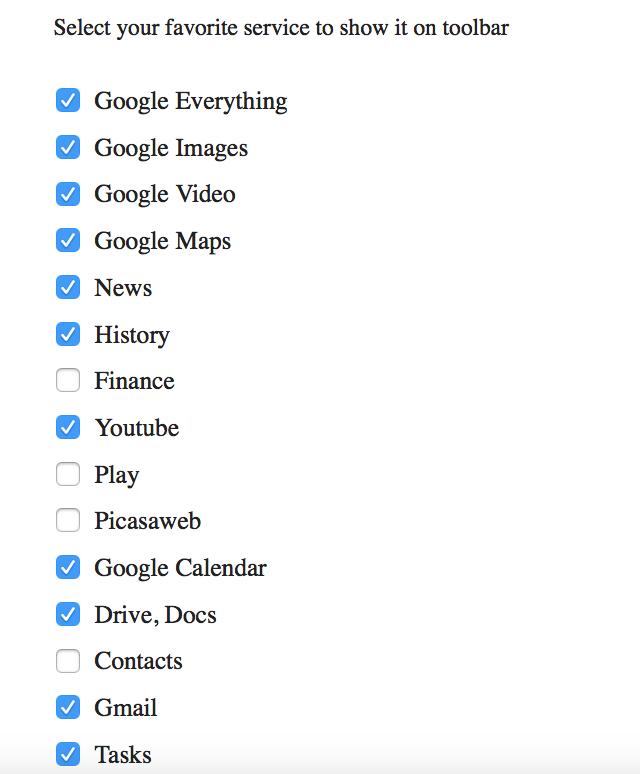The image displays a user interface for selecting services to appear on a toolbar, set against a white background. It features a header in black text that reads "Select your favorite services to show on toolbar." Below the header, a long list of services is presented, each accompanied by a square checkbox.

The services listed include:
1. **Google Everything** (blue box with a white check mark)
2. **Google Images** (blue box with a white check mark)
3. **Google Video** (blue box with a white check mark)
4. **Google Maps** (blue box with a white check mark)
5. **News** (blue box with a white check mark)
6. **History** (blue box with a white check mark)
7. **Finance** (white box, no check mark)
8. **YouTube** (blue box with a white check mark)
9. **Play** (white box, no check mark)
10. **Picasa Web** (white box, no check mark)
11. **Google Calendar** (blue box with a white check mark)
12. **Drive** (blue box with a white check mark)
13. **Docs** (white box, no check mark)
14. **Contacts** (white box, no check mark)
15. **Gmail** (blue box with a white check mark)
16. **Tasks** (blue box with a white check mark)

All service names are stylized with the first letter of each word capitalized.